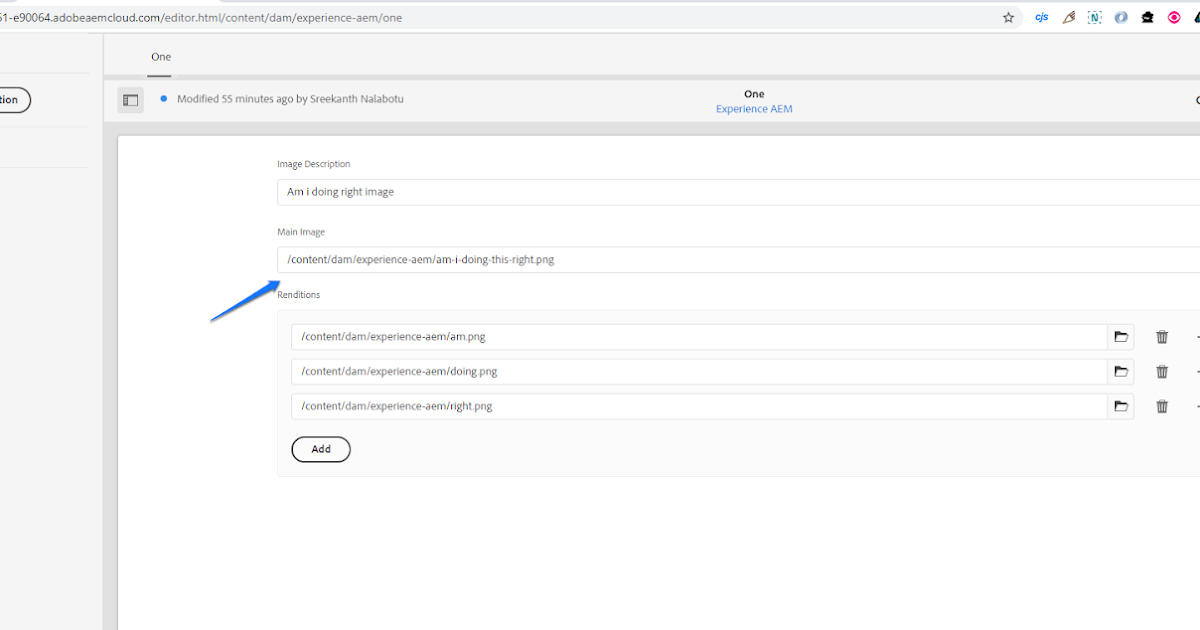**Detailed Image Description:**

The image is a screenshot of some software interface with a predominantly light gray theme. At the top of the screenshot, there is a gray box with the number "1" written inside it, and the number is underlined. Below this, another gray box contains the text "Modified 55 minutes ago by Street Cat, Nalabutu," with the latter part of the text highlighted within a blue circle.

In the middle section of the screenshot, there's the number "1" displayed prominently, followed by the text "experience AEM" in blue letters. All this information is enclosed within light gray boxes, maintaining the theme.

The main portion of the image shows a file path written as `\content\DEM\experience\AEM\am I doing this right.PNG`, clearly annotated with a big blue arrow pointing toward it.

Following this are several renditions of content paths listed as:
1. `\content\DEM\experience-AEM\AEM.PNG` - This line includes an icon of an open folder and a trash can to its right.
2. `\content\DEM\experience\AEM\doing.PNG` - Similarly, this line also features an icon of an open folder and a trash can.
3. `\content\DEM\experience-AEM\right.PNG` - This final rendition line has the same icons of an open folder and a trash can alongside it.

At the very bottom of the screenshot, there is a button labeled "Add," which is encased in a black border.

Overall, the screenshot appears to be highlighting different versions or renditions of content within a digital experience management system, specifically related to Adobe Experience Manager (AEM).